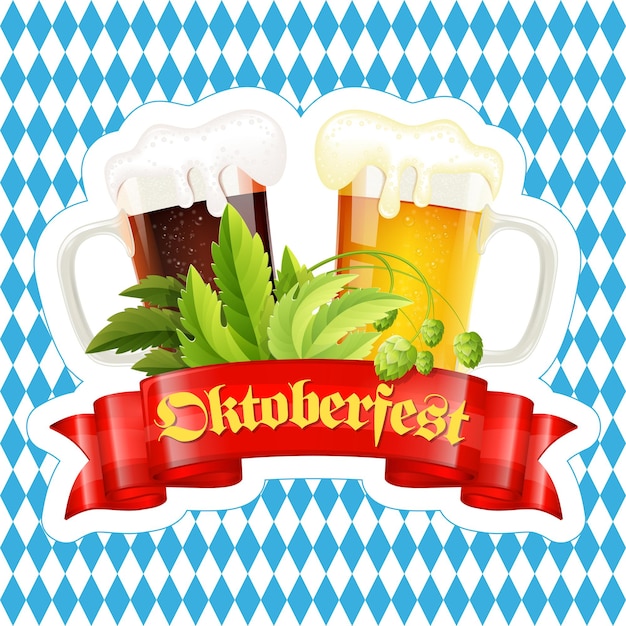This is a detailed computer-animated illustration featuring two overflowing beer mugs. The mug on the left contains a darker beer, reminiscent of a Coca-Cola color, with a foamy white head dripping down its side and its handle pointing to the left. The mug on the right holds a lighter, gold-colored beer with a yellowish head also dripping over the edge and its handle pointing to the right. Both beers are nearly full and feature little white bubbles. Nestled between the mugs are green leafy plants with small buds, likely hops. Below the mugs, a vibrant red ribbon with the stylized gold lettering "Oktoberfest" adds to the festive theme. The background showcases a blue and white diamond checkered pattern, enhancing the celebratory Oktoberfest atmosphere.